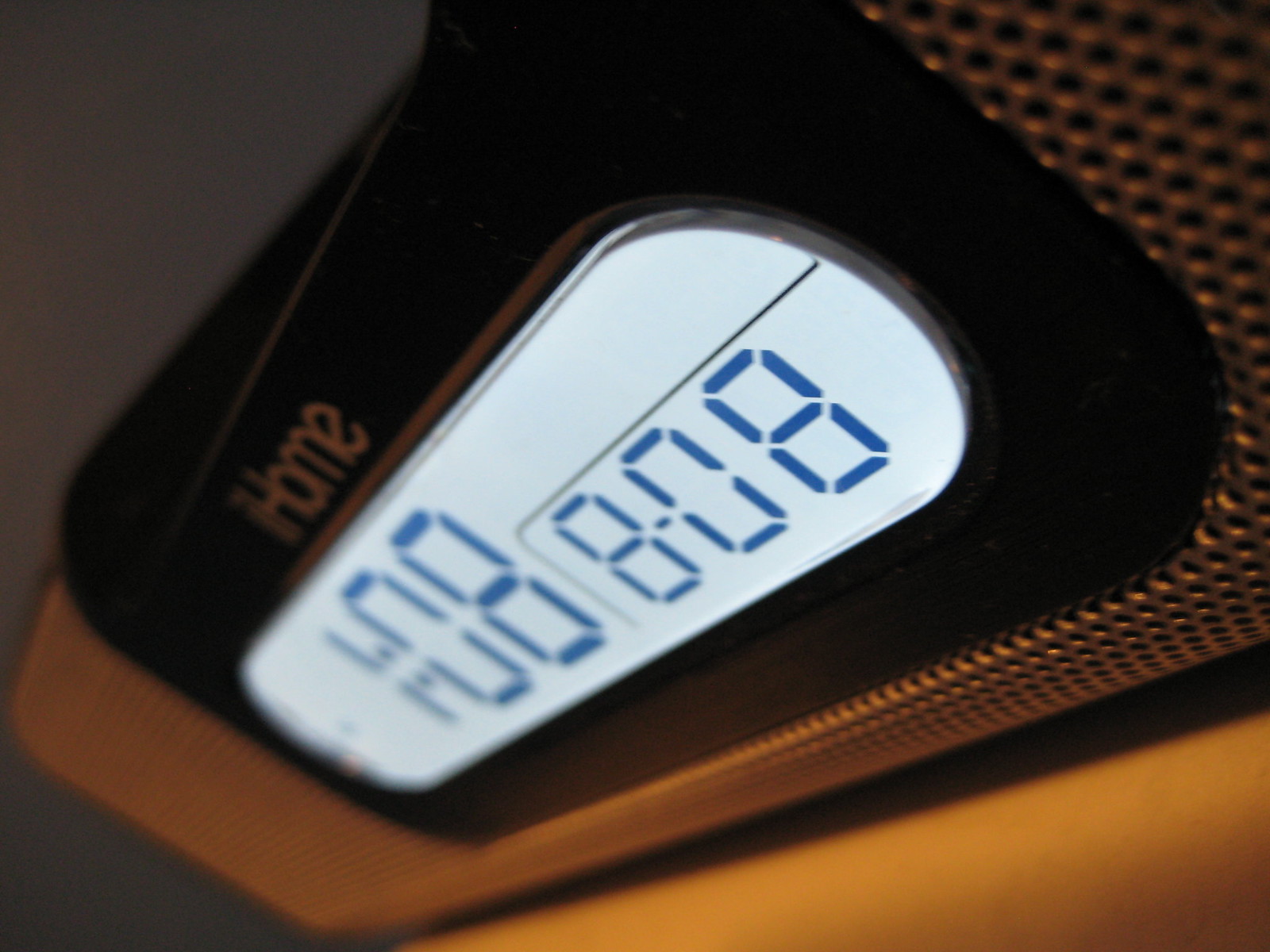This image features a digital alarm clock resting on a light brown table. The photograph is taken at an angle, with the left side of the clock pointing toward the lower left corner and the right side toward the upper right. The clock is branded iHome, and it has an oval-shaped face with a grayish background and black digits. The time displayed is 1:08, and the date in the lower right corner reads 8-08. The front of the clock is black plastic, while a gray-silver speaker area encircles it. The table is light brown, contrasting with the dark gray wall in the background.